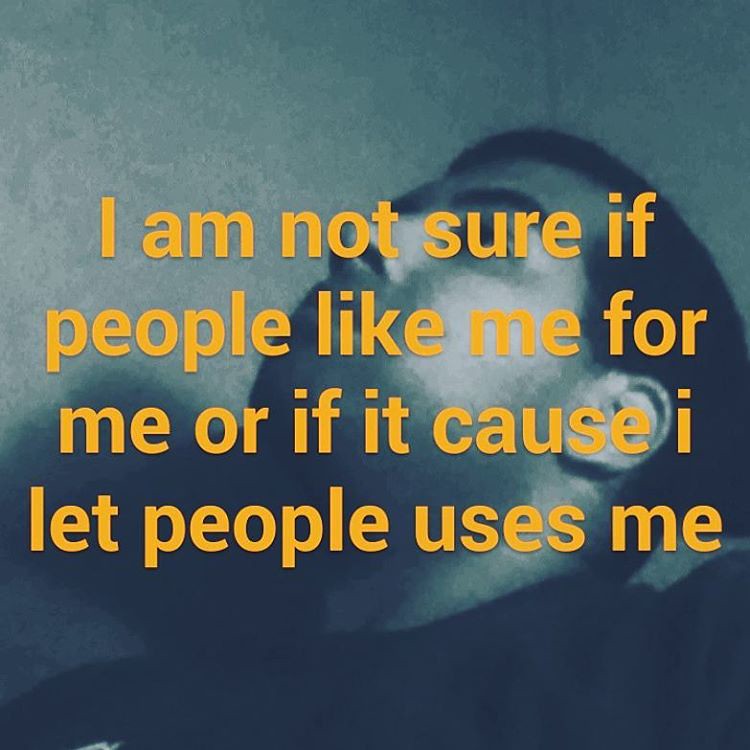The image is a vertically-oriented photo featuring a male with dark, short hair and dark eyebrows, potentially Hispanic. The background is a blurred mix of dark, gray, and greenish-gray shades, appearing sponged or blotchy. The man is depicted lying down or leaning back slightly, possibly with his eyes shut, making the context of his posture ambiguous. He is wearing a dark-colored shirt. Superimposed on the image, in large yellow-orange letters, is the text: "I am not sure if people like me for me or if because I let people uses me." This text stands out against the otherwise muted background, reflecting a sense of uncertainty and self-doubt in the subject's expression.